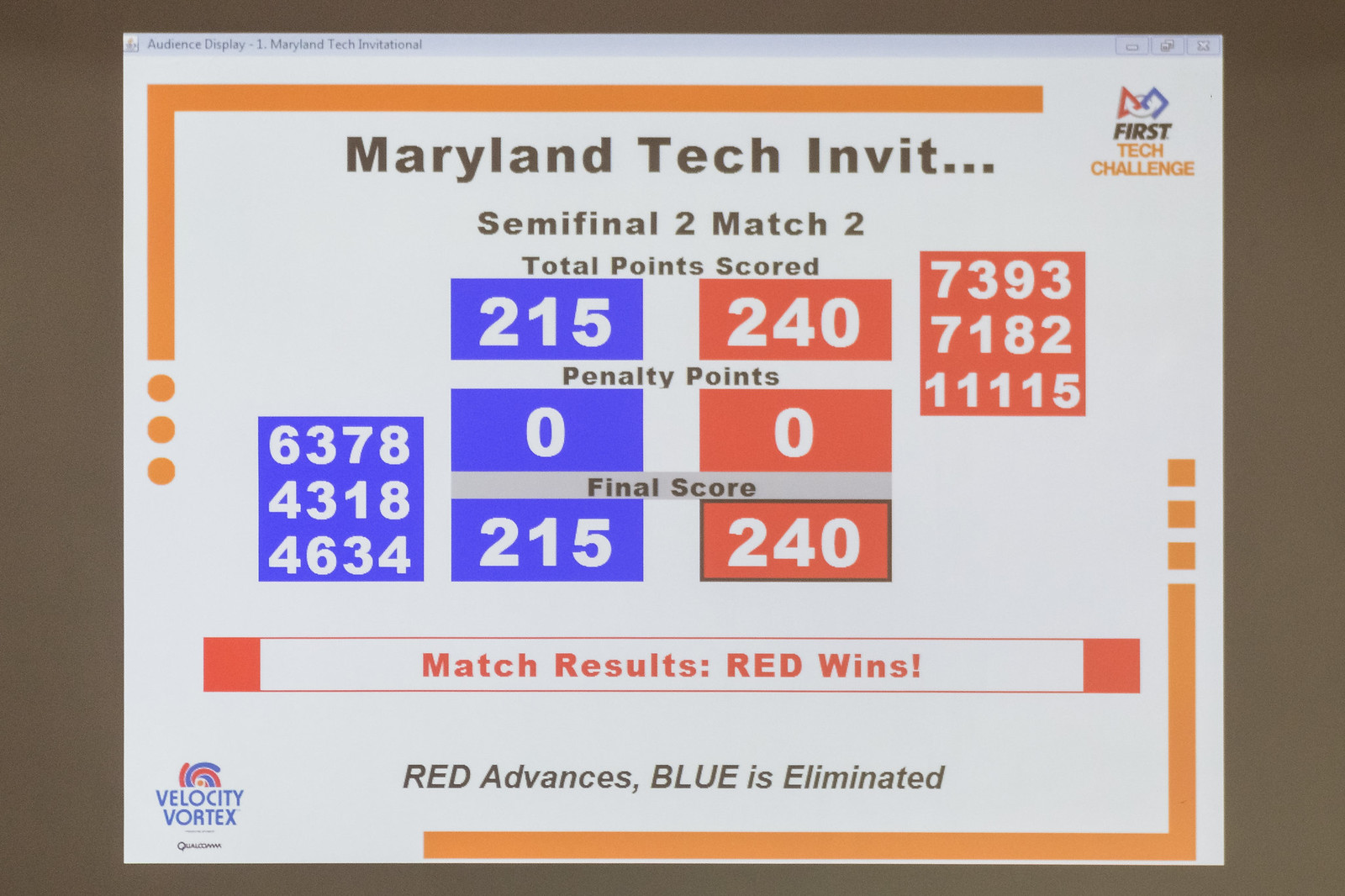This image captures a detailed snapshot of a website displaying the Maryland Tech Invitational’s First Tech Challenge semi-final match two. The page prominently features a scoreboard against an all-black background, with the header reading "Audience Display: Maryland Tech Invitational." Information presented includes the match result: total points scored, 215 for the blue team and 240 for the red team, with zero penalty points for both teams. The final score confirms a red team victory at 240 points. The left side has boxes in blue showing scores and the right side has boxes in red. The words "Match Results: Red wins" are followed by "Red advances, Blue is eliminated," displayed in black text on a gray background. A distinct visual element is an orange frame with three dots on the left and three squares on the right. There's also a small symbol at the top right corner, red and white, and the text "Velocity Vortex" in blue at the bottom left corner. Additionally, the website's URL is not visible, and no time or date is shown in the bottom status bar.